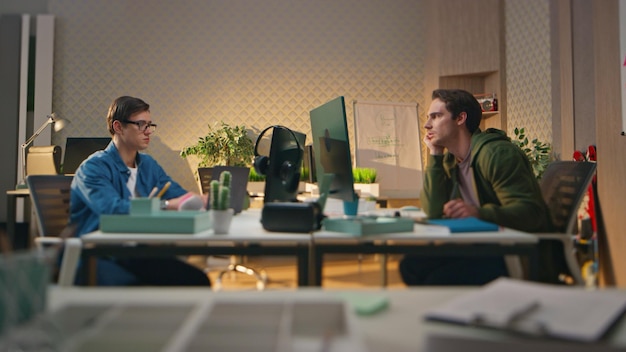In an office environment with a modern, silver-toned desk and chairs, two men are seated opposite each other, each with a laptop in front of them. The desk between them is adorned with various office supplies, including books, light blue desk organizers, a small cactus in a white pot, and several other plants. Both men appear to be deeply engaged in conversation. The man on the left wears glasses and a blue button-up shirt over a white t-shirt, with headphones resting on his computer monitor. The man on the right has a gray shirt with a green hoodie, appearing thoughtful as he rests his head on his hand. 

In the background, a white wall with a textured, hexagonal pattern reminiscent of a golf ball stands out. There are natural wood tones, like a wooden door, adding warmth to the room. Several plants, including a potted green plant and smaller white pot plants, contribute to the room's organic feel. Additionally, there's a built-in corner shelf on the right side, partially obscured by one of the men, and a white banner or paper also occupies that wall space. 

A table lamp on a smaller table, more shelves, and some papers further furnish the room. A blurred foreground suggests other furniture or objects, including what appears to be a red item leaning against the wall, possibly a flag. Overall, the scene is softly illuminated by what could be natural sunlight, adding a gentle ambiance to the office setting.